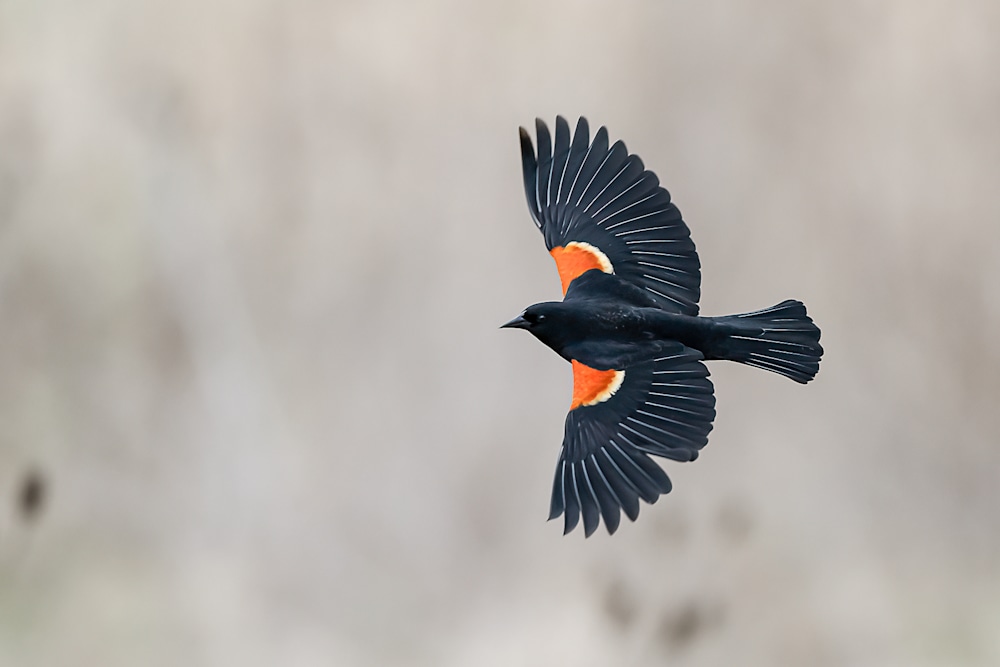The image captures a striking scene of a bird suspended in mid-flight against a blurry, almost faded gray background. The background is indistinguishable except for a few hints of leaves or tree parts, focusing all attention on the bird itself. The bird's body and wings are predominantly black, with wings spread straight up and down as if it's gliding sideways. The most eye-catching feature of the bird is the vibrant orange patch at the top of its wings, accentuated by a white stripe beneath it. Additionally, a black stripe appears at the wings' edges. Its black tail, black beak, and bright eyes add to its distinctive appearance. The bird's precision in flight is emphasized, although one feather on the left wing appears slightly bent. The overall effect is a mesmerizing portrait of a bird gliding effortlessly through the air.